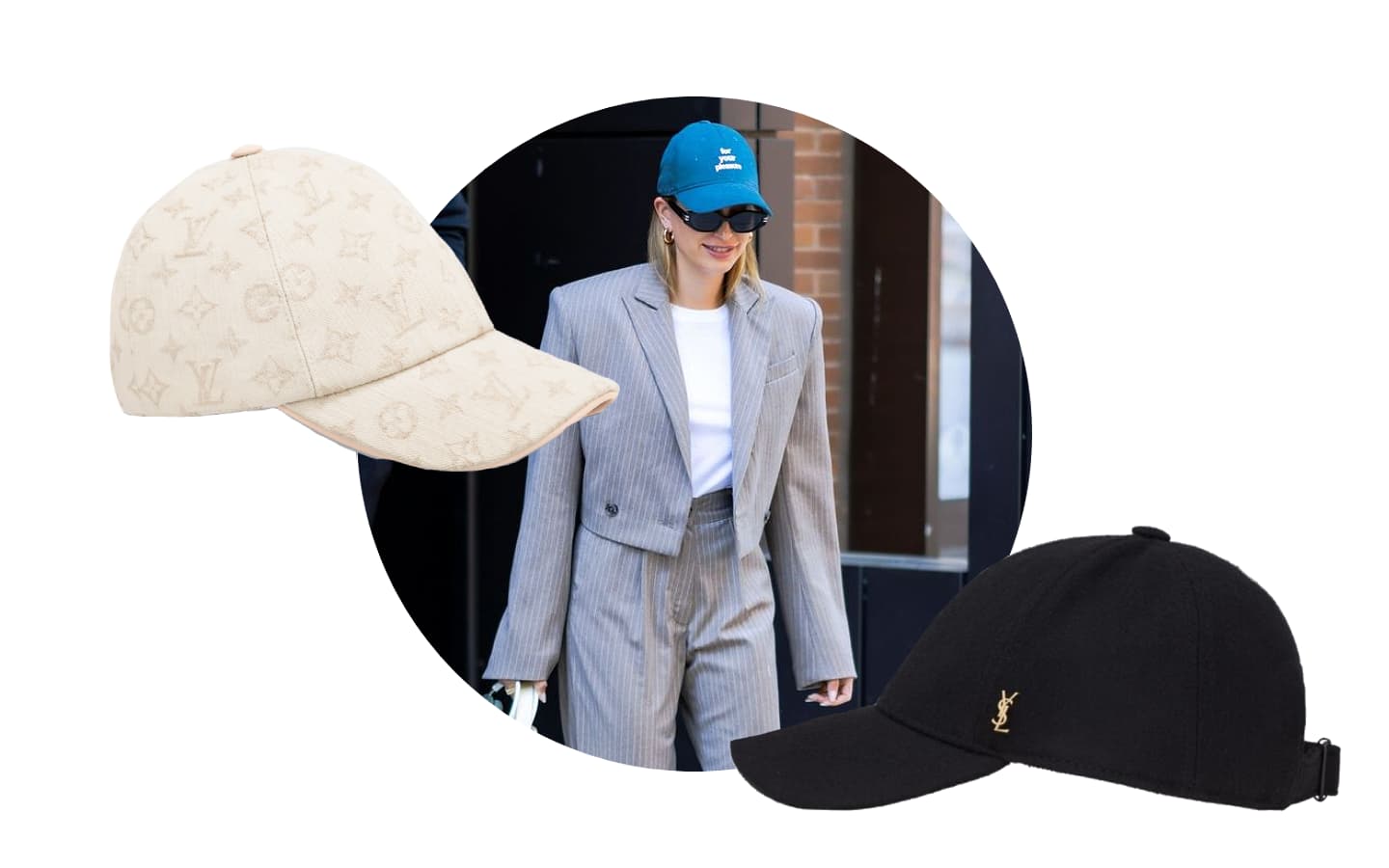The image is a landscape-oriented color photograph featuring a central circular portrait of a young woman, approximately 20 years old, depicted from the top of her head to mid-thigh. She has straight blonde hair and is smiling while looking down. The woman is walking outside against a backdrop of a brick building with a window visible in the background. She is dressed in a subtly striped gray and white suit jacket and matching pants, with a white shirt underneath. She accessorizes with hoop earrings, black sunglasses, and a turquoise blue baseball cap featuring three stacked white words on the front.

Surrounding the circular portrait is a plain white background that creates the illusion that the image and additional elements are floating. To the left of the circle, there is a close-up side view of a cream-colored cap embellished with patterns resembling stars, which some might identify as Louis Vuitton symbols. On the bottom right of the image, another superimposed cap is visible—a black baseball cap featuring a gold designer logo that resembles a dollar sign with a V through it, potentially representing YSL (Yves Saint Laurent). The photograph exemplifies color photographic representationalism, with aspects of both realism and product photography.